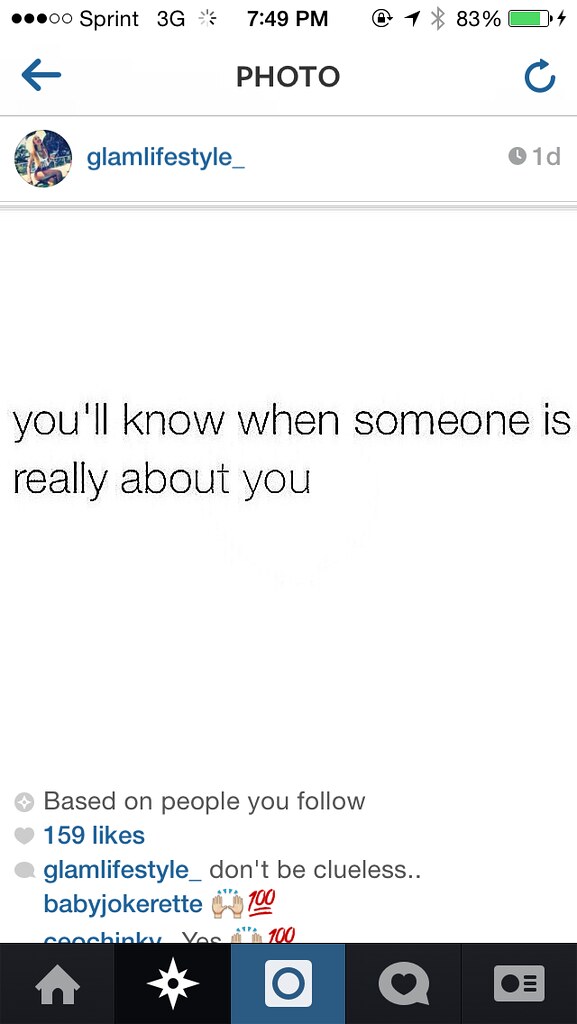The image is a detailed screenshot taken from an older model iPhone displaying an Instagram post, indicated by the Sprint 3G network, at 7:49 PM, with an 83% battery. The top of the screen features traditional iOS icons and text, including a left-pointing blue arrow labeled "photo" in the center, and a blue refresh button on the right. The profile being viewed, identified by a circular profile picture of a woman wearing a hat, belongs to the user "GlamLifestyle_". The post, made one day ago as marked by a small grey clock icon with "1D", consists of a quote on a white background that reads, "You'll know when someone is really about you." The post has garnered 159 likes, highlighted in blue. Below the text, GlamLifestyle_ has commented, "Don't be clueless," followed by responses such as "100%" and "Yes." At the very bottom of the screenshot are traditional Instagram navigation icons: a home symbol, a star, a square icon with a circle, a comment bubble with a heart inside, and a rectangular icon with a circle and three vertical lines.